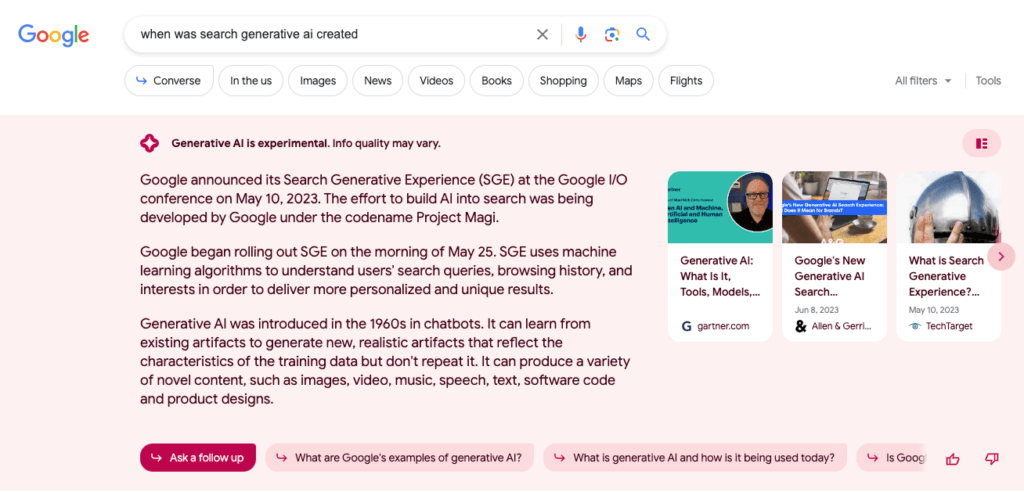A detailed screenshot of a Google search page is depicted. The familiar Google logo is positioned at the top left corner next to the search bar, where the user has entered the query: "when was search generative AI created." Within the search bar itself, there are several icons to the left and right - a microphone symbol for voice input, a small 'X' to clear the search, a camera-like icon for image searches, and the classic magnifying glass that signifies search.

Beneath the search bar, a series of navigational categories are outlined: Converse, In the US, Images, News, Videos, Books, Shopping, Maps, and Flights. Adjacent to these tabs, there are options labeled 'All filters' with a down arrow for additional filtering options, and 'Tools' for further search functionalities.

The search results are presented within a light pink rectangular box, bearing an important notice in a dark reddish burgundy font that reads: "Generative AI is experimental, info quality may vary." The text is relatively small but legible.

Below this notice, the content proceeds to detail: "Google announced the search generative experience (SGE) at the Google I/O conference on May 10th, 2023. The effort to build AI into search was being developed by Google under the code name Project MAGI (M-A-G-I)." The following paragraph notes that: “Google began rolling out SGE on the morning of May 25th. SGE uses machine learning algorithms to understand user search queries, browsing history, and interests in order to deliver more personalized and unique results.” 

Another paragraph provides historical context on generative AI: "Generative AI was introduced in the 1960s in chatbots. It can learn from existing artifacts to generate new, realistic artifacts that reflect the characteristics of the training data but don't repeat it. It can produce a variety of novel content such as images, video, music, speech, text, software code, and product designs."

To the right, there are three relevant images: The first features a headshot of a bald man wearing glasses against a greenish background, captioned "Generative AI, what is it, tools, models." The second image shows someone working on a computer or laptop at a desk, captioned "Google's new generative AI search." The third image depicts a hand spread apart, seemingly gesturing toward something, with the caption "What is search generative experience."

This caption provides a thorough overview of the Google search page, capturing the elements and specific content related to generative AI results displayed to the user.